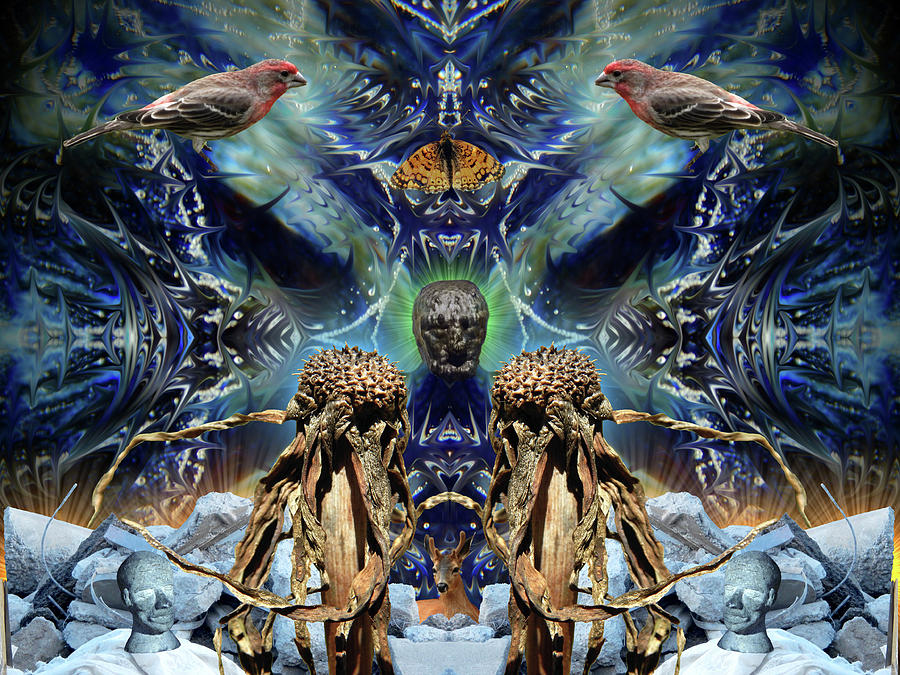The image is a surreal digital artwork featuring a symmetrically intricate design with a tie-dye-like, fractal background in shades of blue, gray, white, and black, suggesting water and feathers. Dominating the scene are mirrored elements including red, black, and white birds positioned on the upper left and right, each with gray beaks. An orange and black butterfly or moth flutters at the top center. Beneath the birds, at the lower left and right, are brown objects resembling dead plants or dried flowers. In the central portion of the image is a gray rock with a face, its eyes and mouth black, and shoulders and neck highlighted in blue. Flanking this central rock are black statues seated on gray rocks, adding to the mythological ambiance. Additionally, a deer stands prominently in the middle bottom section, characterized by its brown color and distinctive black eyes and nose. The entire composition exudes a striking blend of natural and fantastical elements with hints of machinery and robotic forms interspersed throughout.